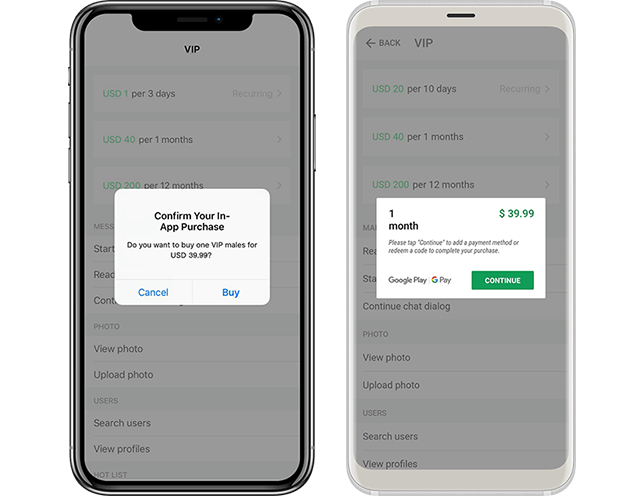The image is a screenshot displaying two smartphones positioned side by side, each showcasing a pop-up window. Both smartphones are identical in height and width and possess grayed-out backgrounds, which allows the text on the phones to remain visible despite the dull backdrop. The phone on the left features a gray frame, whereas the phone on the right is framed in white.

On the left phone, the pop-up window is white with rounded corners. The text within this window reads, "Confirm your in-app purchase. Do you want to buy one VIP meal for USD 39.99?" This is written in black text. Below this prompt, there are two blue options: "cancel" on the left and "buy" on the right.

The phone on the right also displays a white rectangular pop-up window. In the upper right corner of this window, "39.99" is written in green text. Directly below this, a green "continue" button is prominently featured.

Despite their similarities in structure and layout, the pop-up windows on each phone provide slightly different designs and prompts for the in-app purchasing process.